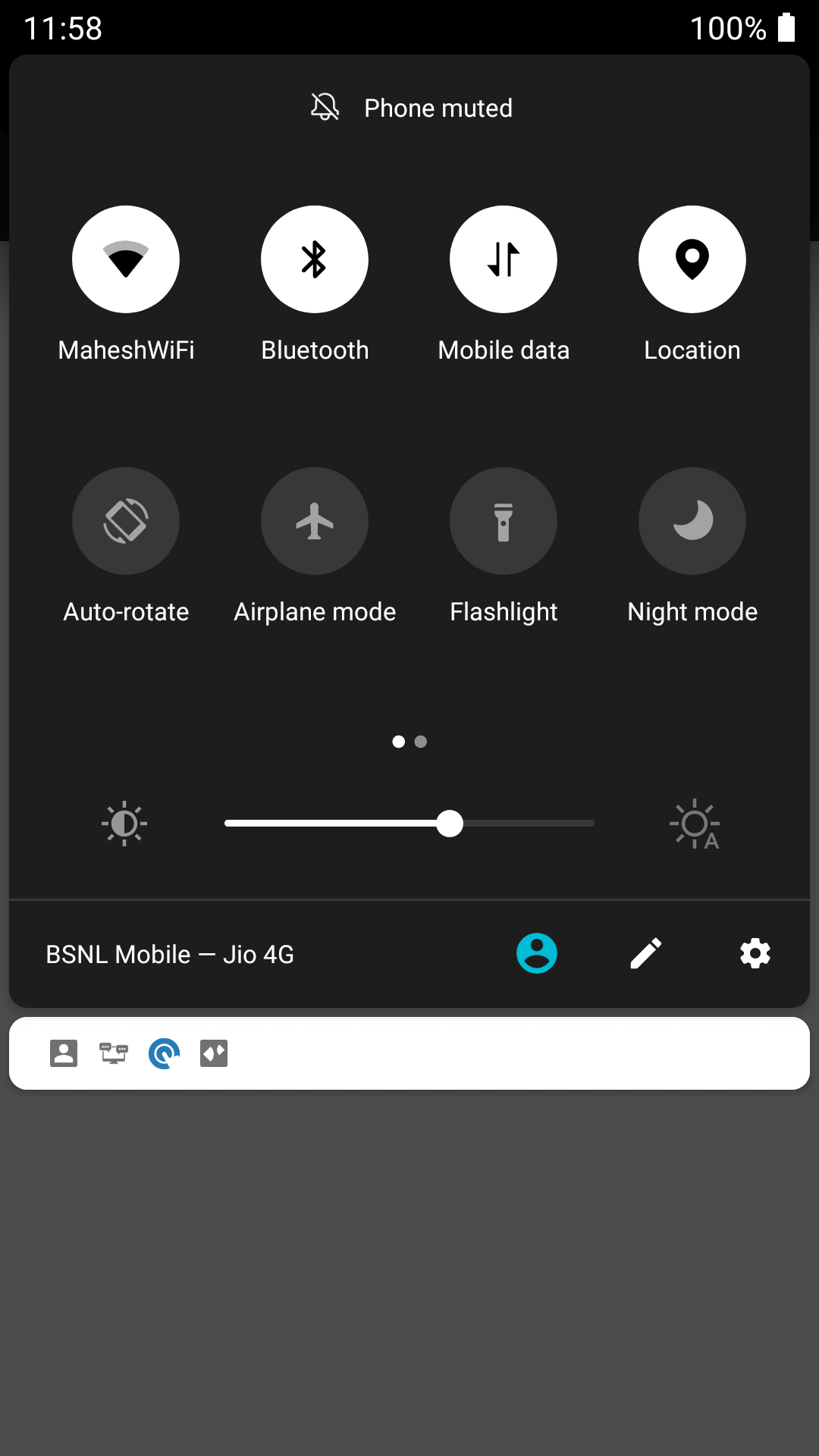This is a detailed description of a mobile phone screenshot displaying the device's control center in dark mode. The background is a deep charcoal black, and there's a darker black bar at the top. In the left corner of the top bar, the time reads "11:58," and in the right corner, a battery icon displays "100%" along with the text "Phone muted" and an icon of a bell with a slash through it.

Immediately below this top bar, there are various settings icons arranged in white circles. From left to right, they include "My Wi-Fi," "Bluetooth," "Mobile Data," and "Location." Beneath these are additional settings in gray circles: "Auto Rotate," "Airplane Mode," "Flashlight," and "Night Mode."

Further below, there is a brightness adjustment slider. Beneath the slider, in white font, it says "BSNL Mobile - JIO 4G." Adjacent to this text, there's a blue circle with a black silhouette of a human, a pencil icon, and a gear icon.

Below this section, there is a white rectangle containing four icons: a gray square with a white human silhouette, a computer monitor icon, a blue half-circle icon, and another gray square with a small white diamond in it. At the bottom of the screenshot, there is a large, empty gray rectangle.